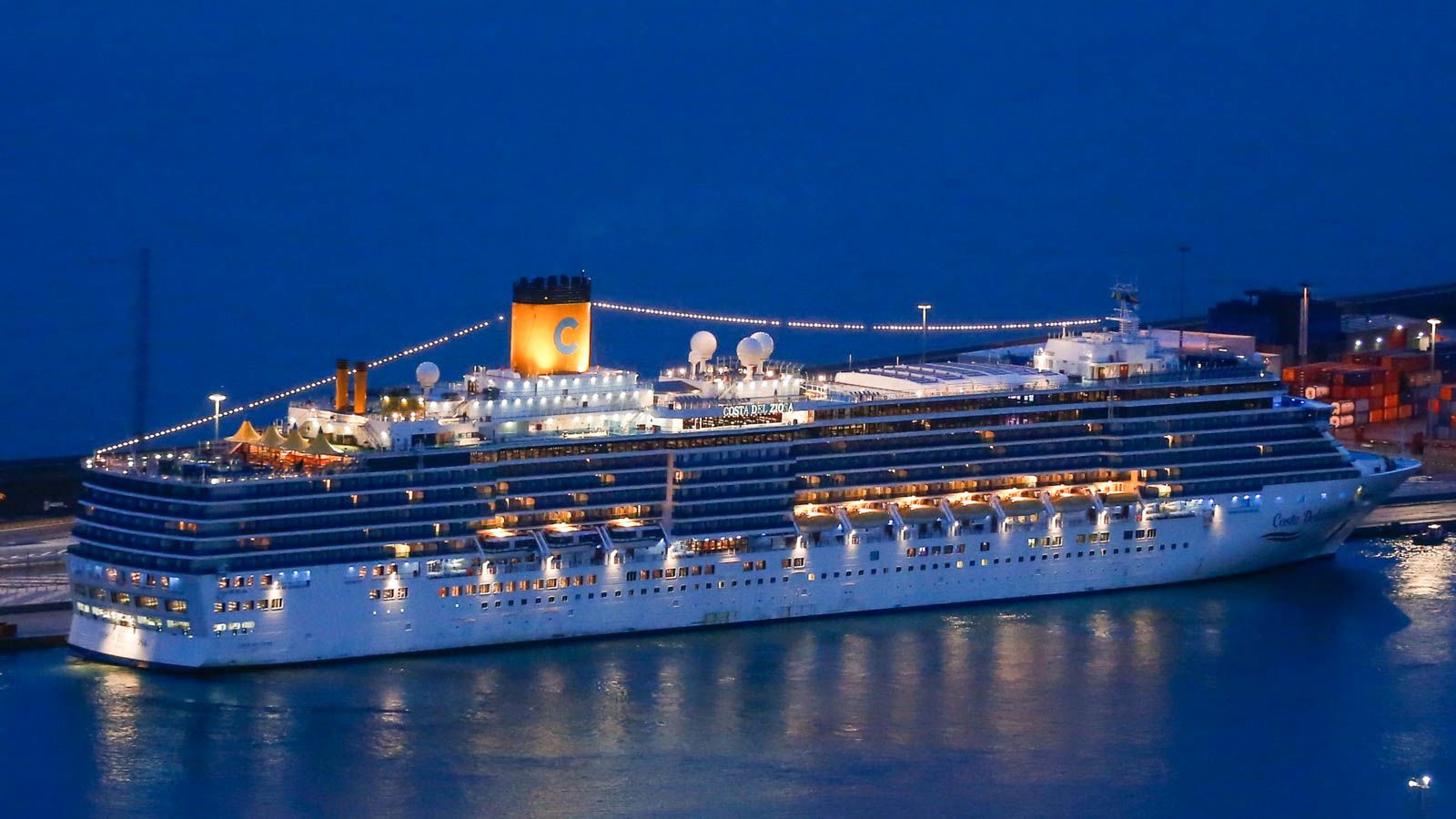In this faraway nighttime photograph, a huge cruise ship adorned in blue and white dominates the scene, creating a striking contrast against the dark blue sky and glistening water. The ship is brightly lit from bow to stern, with many windows and porthole windows glowing warmly. Central to the ship, there is a prominent burnt-orange smokestack bearing a 'C' on its side, surrounded by a cluster of circular towers. Smaller black smokestacks and brown ones towards the bow also dot the ship's profile. The top of the ship is lined with a strand of lights, adding to its festive illumination. The water gleams with reflections from these lights, enhancing the grandeur of the scene. On the right-hand side of the background, stacks of cargo containers suggest the ship is docked near a bustling city pier, yet the exact location remains unknown.